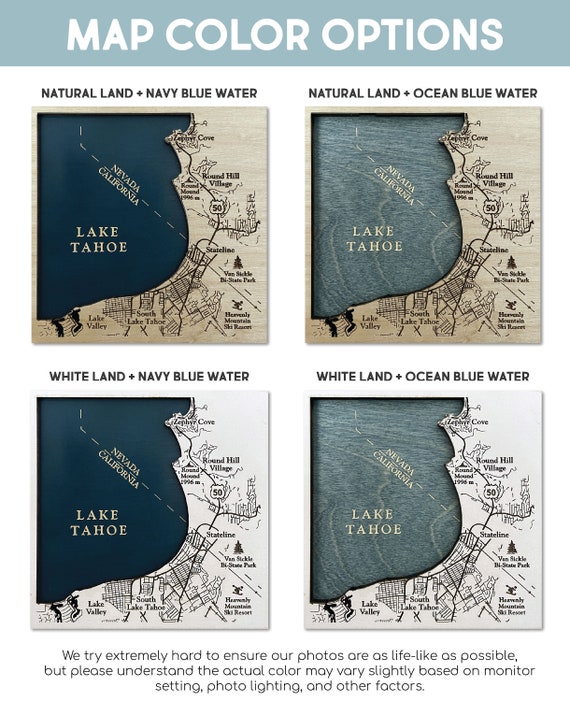The image depicts a vertical collage of four maps showcasing the southeast shoreline of Lake Tahoe, highlighting the border between Nevada and California. At the top, a blue bar with white text labels the section as "Map Color Options." Each map is labeled and organized in a grid of two rows and two columns. The top left map displays "Natural Land & Navy Blue Water," while the top right shows "Natural Land & Ocean Blue Water." The bottom left map features "White Land & Navy Blue Water," and the bottom right exhibits "White Land & Ocean Blue Water." Each map includes landmarks such as Zephyr Cove, Round Mound, Round Hill Village, Interstate 50 State Line, Van Sickle Bi-State Park, Heavenly Mountain Ski Resort, Lake Valley, and South Lake Tahoe. The colors used in these maps are shades of blue, black, beige, white, gray, and light blue. A note at the bottom emphasizes that while efforts are made to ensure the photos are lifelike, actual colors may vary slightly due to monitor settings, photo lighting, and other factors.